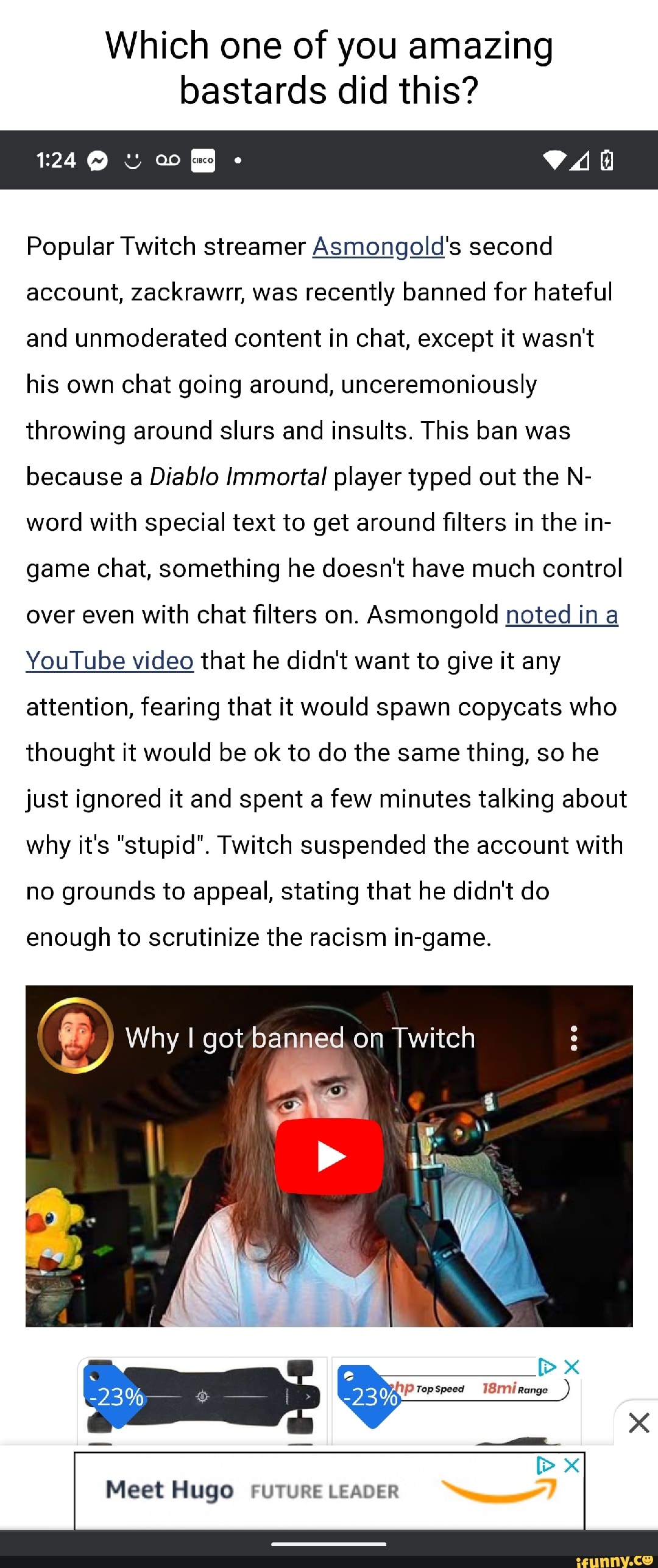The image is vertically rectangular, resembling a smartphone screenshot adorned with text overlays. At the top, a caption reads, "Which one of you amazing bastards did this?" Directly underneath, a horizontal black banner displays the time as 1:24 and includes icons for Messenger, voicemail, Wi-Fi signal, and battery status.

Below this banner, a portion of an article appears, accompanied by a YouTube video thumbnail. The thumbnail, intended to be tappable, features the title, "That's why I got banned on Twitch." This visually engaging screenshot combines humorous commentary with multimedia elements, illustrating a moment likely shared on social media.